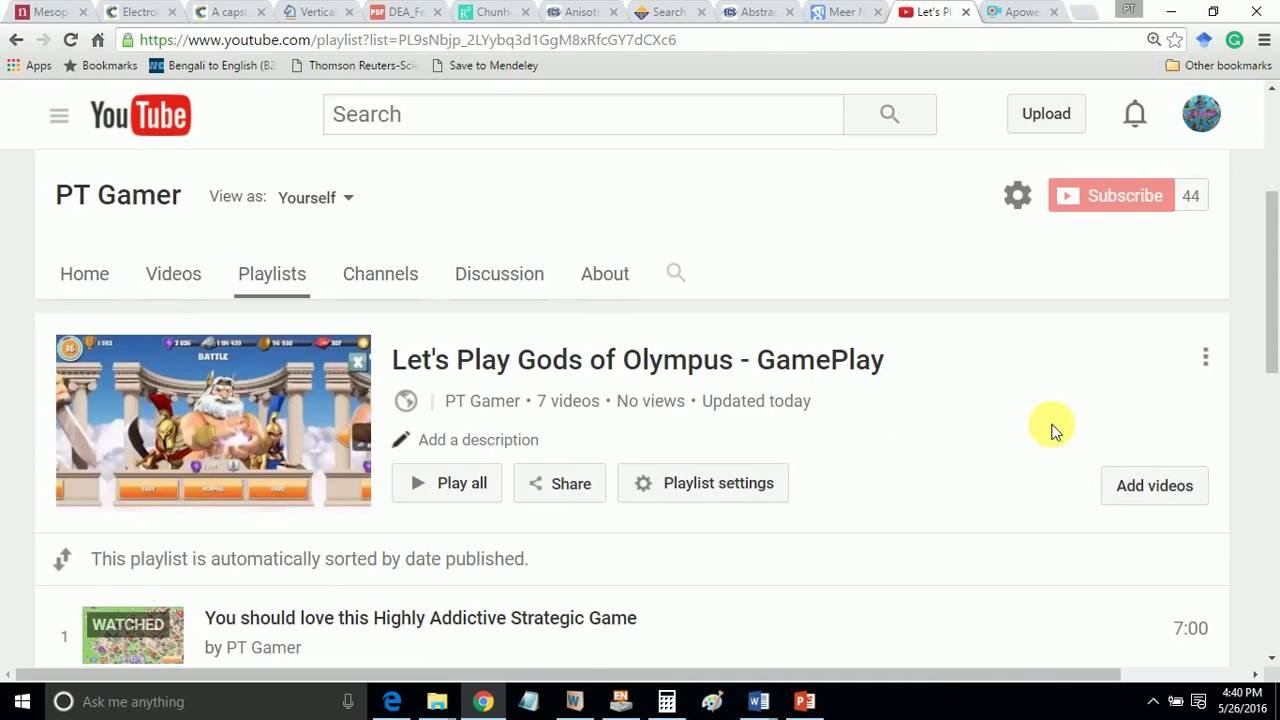This image shows a screenshot of a YouTube channel page belonging to a user named PT Gamer. The browser window is cluttered with multiple tabs, but the YouTube tab is currently active. The main section of the page highlights the "Playlist" tab, which is underlined, indicating it is currently selected among other options such as Home, Videos, Channels, Discussion, and About.

As we delve further into the details, the playlist includes a video titled "Let's Play Gods of Olympus," labeled under the Gameplay category. Accompanying the video title is a thumbnail image featuring a bearded character with golden wings near his head. The character sports a long, white beard and mustache, and he stands in front of classical architecture, under a bright blue sky dotted with scattered white clouds.

Below the video, there is a section that prompts the user to "Add Description." Further details about the channel indicate that PT Gamer has uploaded seven videos, which currently have no views. The page notes that the content was updated today.

A yellow circle can be seen on the screen, highlighting the cursor, depicted as a white arrow, which points at a specific area within the screenshot, drawing attention to the interactive elements of the page.